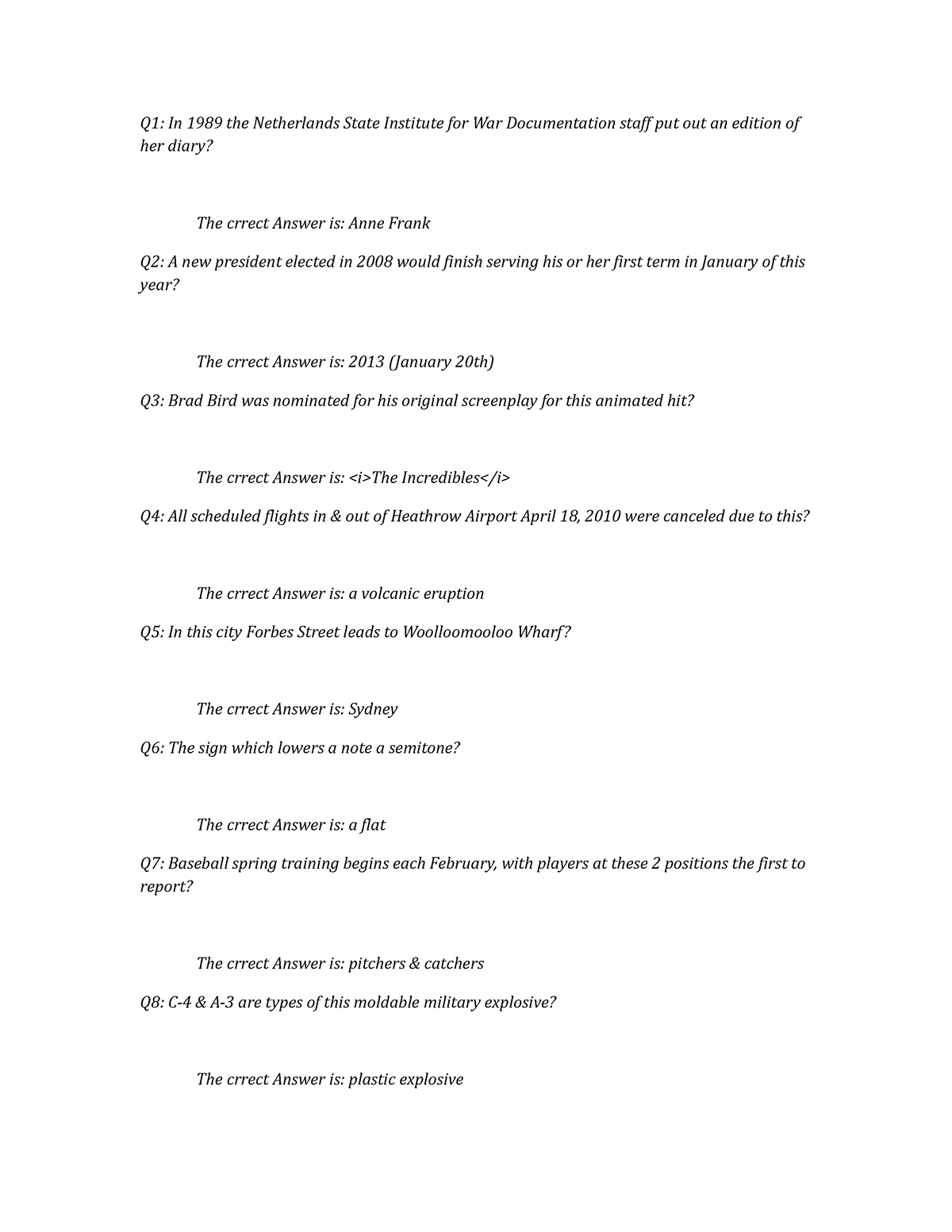Here is the cleaned-up and detailed caption for the image:

---

This is an answer key for a history quiz, presented entirely in italicized font resembling either Georgia or Times New Roman. The formatting and content are as follows:

1. The first entry is labeled as "Q1:" and reads, "In 1989, the Netherlands State Institute for War Documentation staff put out an edition of her diary?" The space following the question holds the correct answer: "Anne Frank."

2. The second entry is labeled as "Q2:" and states, "A new president elected in 2008 would finish serving his or her first term in January of this year?" The correct answer is noted after a space: "2013 (January 20th)." Notably, the word 'correct' is misspelled as "C-R-R-E-C-T," missing the 'O'.

3. The third entry, labeled "Q3:," asks, "Brad Bird was nominated for his original screenplay for this animated hit?" The provided answer is "The Incredibles," which is indicated with an attempt at HTML-style italicization: "<i>The Incredibles</i>."

4. The fourth entry is marked "Q4:" and queries, "All scheduled flights in and out of Heathrow Airport on April 18, 2010, were canceled due to this?" The answer is stated as "a volcanic eruption."

5. The final entry, "Q5:," reads, "In this city, Forbes Street leads to Woolloomooloo Wharf?" Following the characteristic space, the correct answer is given as "Sydney."

---

The quiz key includes typographical attempts to italicize which are inconsistently done, and there are occasional minor errors in spelling and formatting.